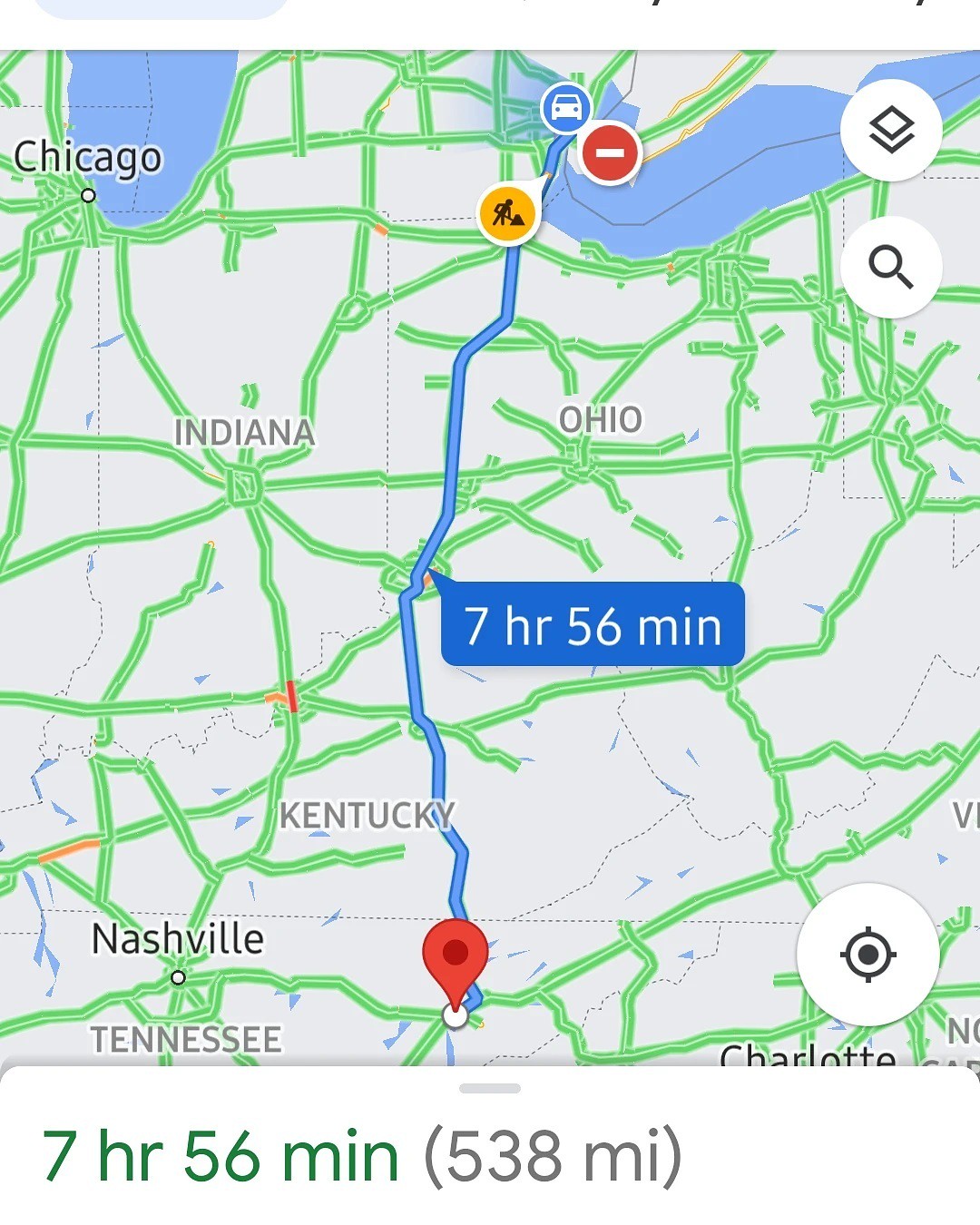Screenshot of a Google Maps navigation route: The image depicts a Google Maps navigation screenshot from a mobile device, showcasing a network of green lines representing major highways and roads crisscrossing several states. Prominent among these states are Indiana, Ohio, and Kentucky, while in the top left corner, the city of Chicago is discernible. Blue areas on the map indicate significant water bodies, most likely Lake Michigan and Lake Erie. Toward the bottom of the map, the states of Tennessee and adjoining regions are visible. A red marker, symbolizing the destination, is situated roughly between Nashville, Tennessee, and Charlotte, North Carolina. The starting point is marked with a blue car icon at the top end of a blue route line, though it is unnamed. An information box within the map indicates the travel time as 5 hours and 56 minutes, covering a distance of 538 miles.